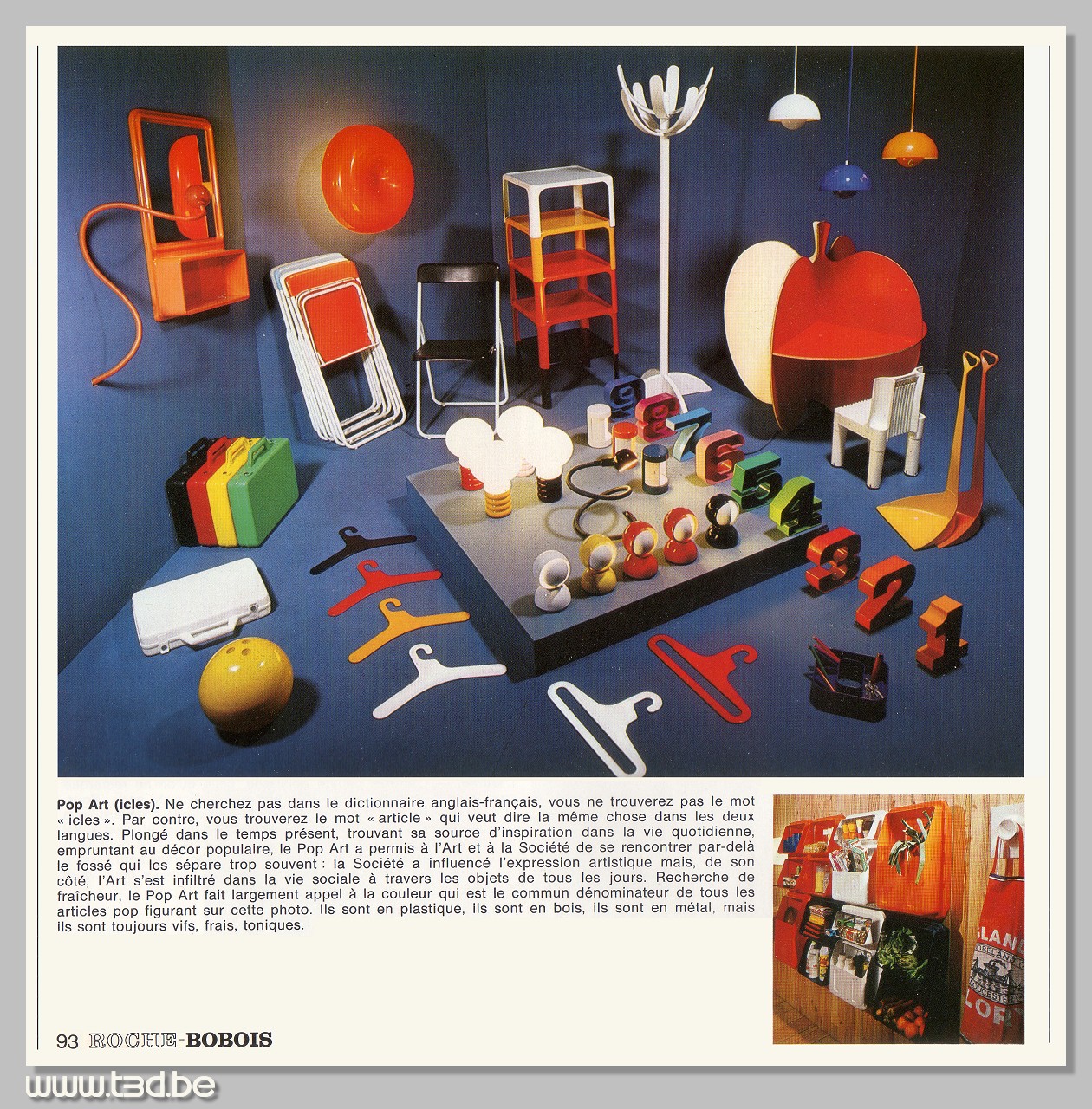The image depicts a vibrant, blue-walled and blue-floored room filled with a dynamic display of pop art items reminiscent of the 70s. The scene is packed with miscellaneous, brightly colored items. Prominent features include hanging lamps in white, blue, and orange; white stacking tables and folding chairs; and brightly colored stacking chairs. On the wall hangs an orange plastic walk, while the floor displays modern art coat hangers in black, red, yellow, and white. 

Various items such as green, yellow, red, and black plastic briefcases are stacked together, with a white suitcase placed nearby. A vivid yellow bowling ball stands out among the clutter on the floor. An eye-catching feature is a circular table that resembles an apple, accompanied by a small white chair, designed as a children's table. Scattered around are the numbers one through nine, seemingly made of plastic, with one through three on the floor and four through nine on an elevated surface among various twist lamps and light bulbs with bright-colored bases. Small orange and yellow shovels add to the colorful array.

Below the image, there is a paragraph written in French with a header that reads "Pop Art I-C-L-E-S." The bottom left corner displays "page 93 Roche-Boubois," and a website "www.t3d.be" is noted. Another image of unknown trinkets hangs on the wall, along with a little apron completing this artistic, eclectic ensemble.